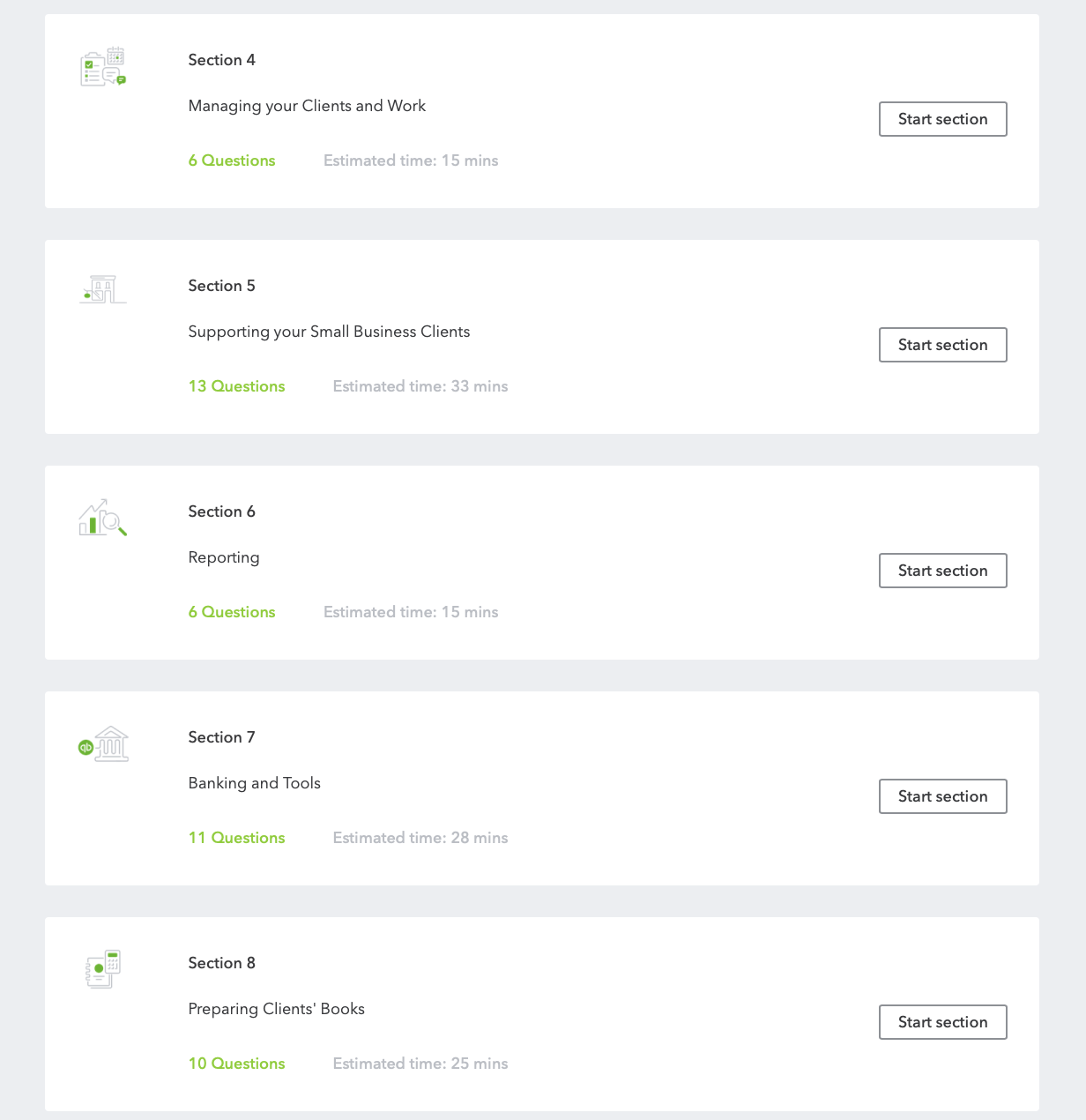The image depicts a clean and minimalistic interface of an online training module. The background is light gray, over which wide, white rectangular panels are arranged vertically. Each panel represents a section of the training course, featuring clear and succinct details about the content within.

At the top, the first panel is labeled "Section 4: Managing Your Client and Work." This section includes an illustration of a clipboard, a calendar, and a phone, suggesting practical tools for client management. It comprises six questions with an estimated completion time of 15 minutes. A search section is also mentioned, perhaps for navigating within the module.

The second panel is labeled "Section 5: Supporting Your Small Business Clients." This section contains 13 questions and has an estimated duration of 33 minutes.

Continuing downward, "Section 6: Reporting" includes icons of graphs and a magnifying glass, indicating a focus on data and analysis. This section has six questions and is projected to take 15 minutes.

"Section 7: Banking and Tools" is next. The iconography here features a building with pillars, evoking stability and structure, likely related to financial management. It has 11 questions with an estimated time of 28 minutes.

The final section visible is "Section 8: Preparing Clients' Books." Symbols like a calendar, a calculator, and what appears to be a ledger suggest financial record-keeping. This section involves 10 questions, estimated to take 25 minutes.

Each panel includes a prominent "Start Section" button on the right, facilitating easy navigation.

At the top, there is a logo depicting a building with a lamp or a green element, although the exact details are unclear. No additional branding or information is provided to indicate the course provider or the specifics of the module. The overall design is sleek and straightforward, aiming to provide a user-friendly experience for learners engaging with the training material.